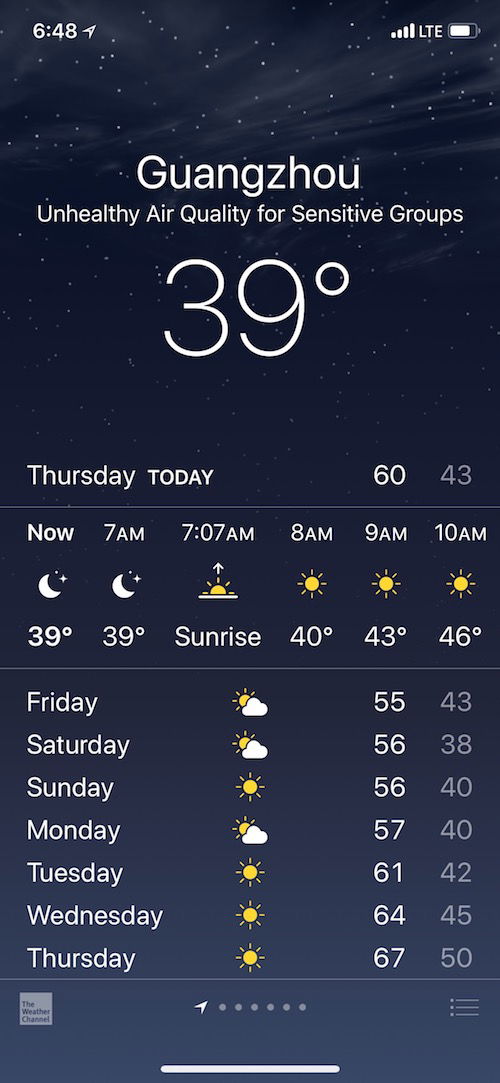**Detailed Screenshot Description:**

The screenshot captures the interface of a weather application on a smartphone, providing intricate weather details for Guangzhou. At the top left corner of the screen, the time is displayed in white font, reading "6:48". In the upper right-hand corner, the screen shows the signal strength bars, the letters "LTE", and the battery icon, indicating the phone's connectivity and battery status, respectively.

The background of the app is dark with star-like patterns, suggesting it is nighttime. At the center top of the screen, "Guangzhou" is displayed in white font, indicating the location for which the weather information is provided. Below this, a warning is displayed in white font: "Unhealthy air quality for sensitive groups." The current temperature is prominently displayed in bold white font as "39 degrees."

Further down, the screen indicates today's date with "Thursday, today." To the right of this, two temperatures are listed: "60" in white font and "43" in gray font, possibly representing the high and low temperatures for the day.

Below this, there are two gray lines, and between them is an hourly weather forecast. This section starts with "now" followed by sequential times: "7 a.m.", "8 a.m.", "9 a.m.", and "10 a.m." Icons next to these times represent the weather conditions, starting with a moon icon, transitioning to a moon partially emerging, and then changing to a sun icon from 8 a.m. onward, indicating the time of day and expected weather.

Another gray line separates this section from the seven-day forecast underneath. Days of the week from "Friday" to "Thursday" are listed in white font on the left-hand side, each accompanied by respective weather icons. The icons indicate weather conditions, such as partly sunny and sunny. Corresponding temperatures are displayed in white for the highs and gray for the lows.

At the very bottom of the screen, on the left-hand side, there is the Weather Channel logo. In the center is the location services icon with a series of dots, and on the far right, a menu option is present, completing the app's interface.

This descriptive caption aims to convey all the details visible in the screenshot comprehensively.